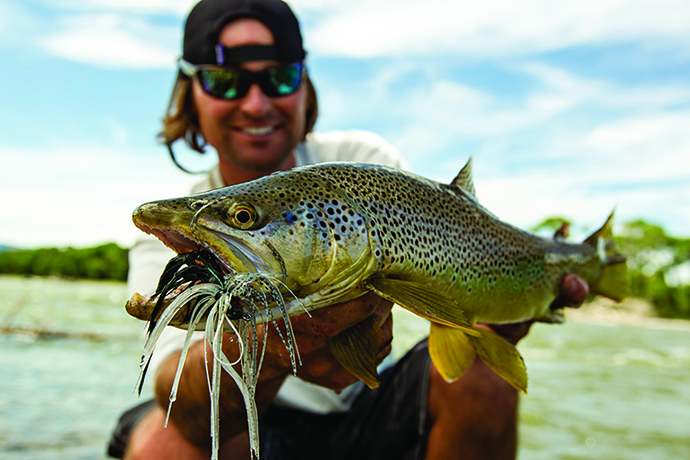The image captures a man, slightly out of focus but visibly smiling, holding a large fish with a lure in its open mouth. The fish, positioned centrally and in sharp focus, boasts a silvery-brown body adorned with numerous black spots, with yellow fins and striking yellow eyes. The man is wearing reflective black sunglasses, a backwards black baseball cap, and has long brown hair trailing just below the cap. He sports a white t-shirt and dark shorts, and appears to be either sitting or kneeling near a waterbody, likely a river or large lake. The background reveals a serene scene with green trees lining the riverbank and a partly cloudy sky adding splashes of blue amidst the white.